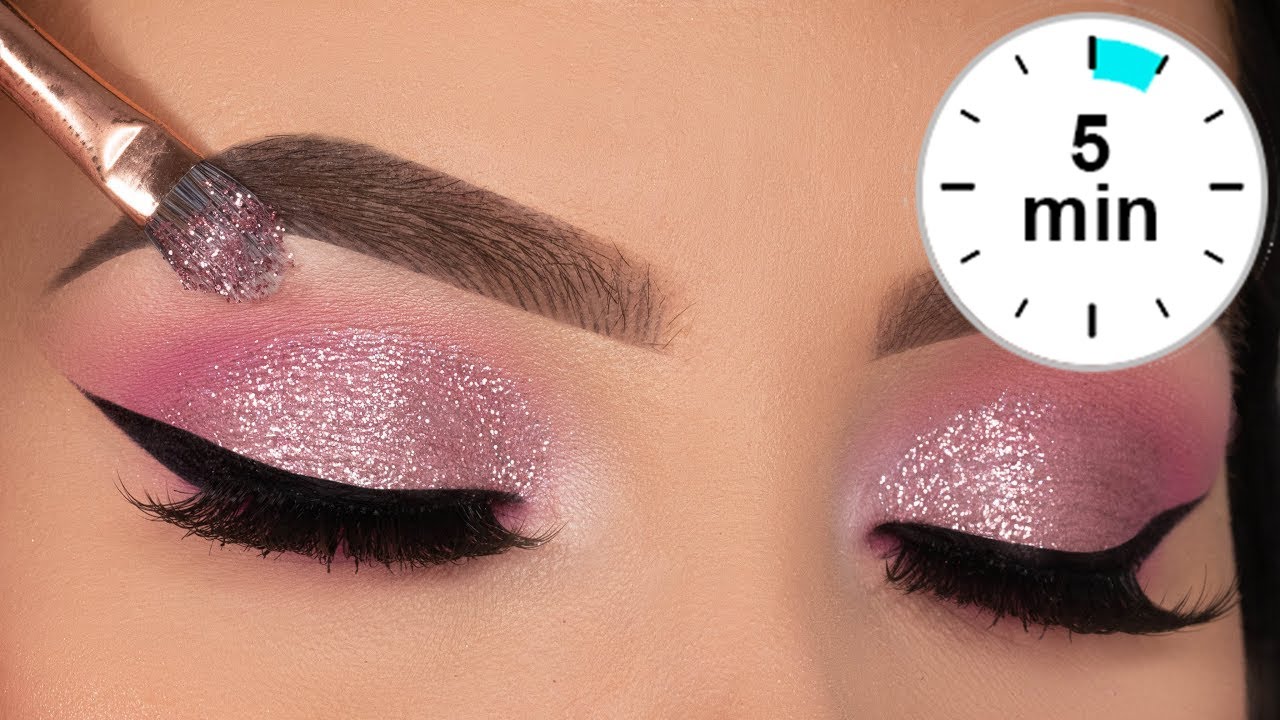The image depicts an up-close view of a woman's closed eyes, showcasing an elaborate eye makeup application. Her skin is light, smooth, and porcelain-like, with no visible pores. The eyebrows are highly defined, likely enhanced through microblading, and are brown in color. The striking eye makeup features a pink, silver, and purple shimmery eyeshadow that has been meticulously blended across the eyelids, which are closed. A thick, black winged cat-eye eyeliner accentuates the upper lids, accompanied by voluminous false lashes. A makeup brush, laden with matching sparkly pink eyeshadow, is seen in the top left corner, indicating its recent use in applying the makeup. In the top right corner of the image, a white clock with a teal indicator prominently displays "5 minutes," suggesting the duration of the makeup application or a step in a makeup tutorial. The overall impression is of a highly detailed, possibly instructional, snapshot of a makeup ad or tutorial.